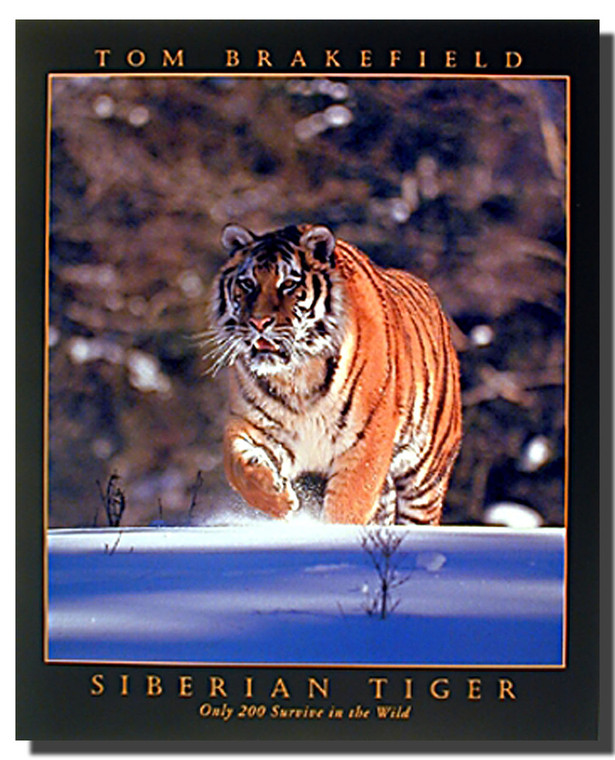The image appears to be the cover of a book with a black background. At the top, in bold gold print, is the author's name, "Tom Brakefield." Below this, a large rectangular area bordered by a thin gold frame contains the striking image of a tiger. The tiger, orange with black stripes, white above the eyes, a pink nose, and a white underside and whiskers, is captured facing forward with an open mouth and piercing eyes as it walks through the snow. The snowy foreground has a few pieces of grass sticking up, while the blurred background suggests a forest of leafless trees. At the bottom of the image, in gold print, the words "SIBERIAN TIGER" are prominently displayed, followed by a sobering note in smaller print: "Only 200 survive in the wild." This striking visual and poignant caption highlight the rarity and magnificence of the Siberian tiger, emphasizing its endangered status.